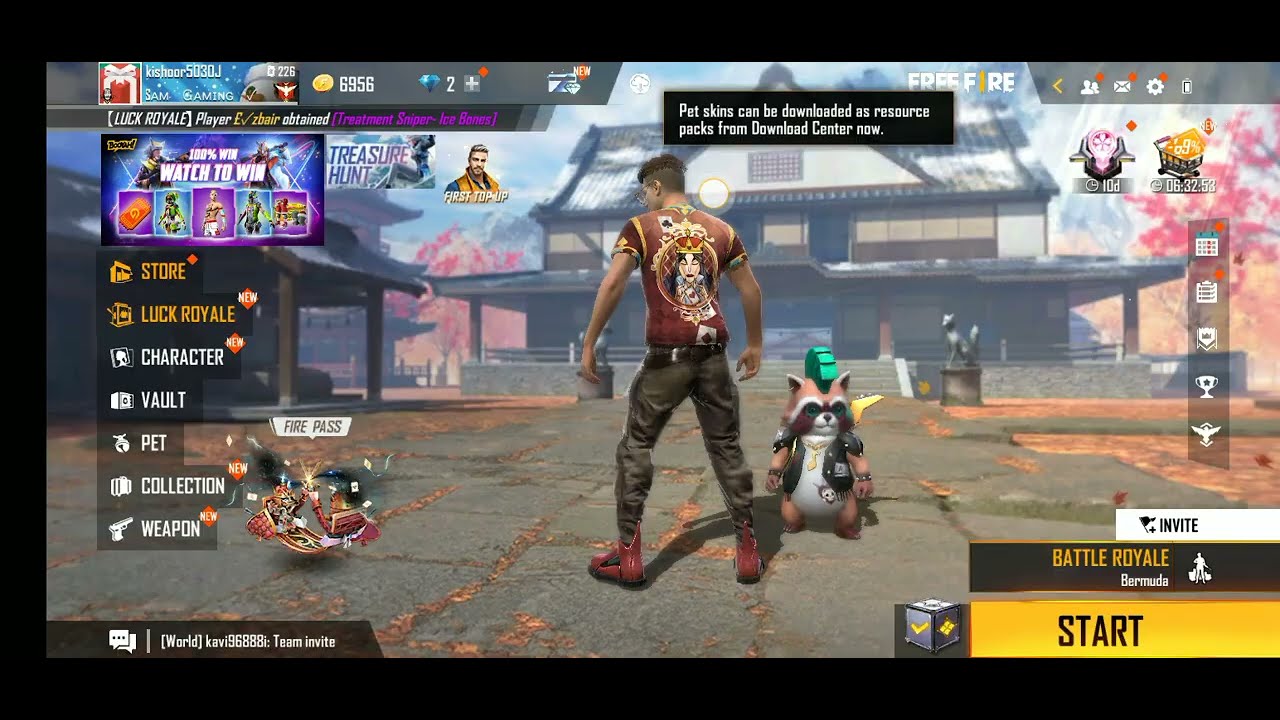In the screenshot of a video game, possibly Overwatch or Fortnite, we observe a detailed and bustling main screen. At its center is a character with a brown shirt featuring a design of a woman wearing a golden crown, accompanied by playing cards adorned with black spades and clubs. The character, who has brown hair and glasses, is also dressed in gray pants and distinctive red boots. Nearby, on the right side, stands a raccoon with a green mohawk, sporting a small leather jacket and a yellow tie, adding a quirky touch to the scene.

The game's user interface is rich with information. The top section displays messages indicating that pet skins and resource packs can be downloaded from the download center. Various menu options are prominently shown, including Store, Luck Royale, Character Vault, Pet, Collection, and Weapon. Other features of the interface include Fire Pass, Team Invite on the bottom left, and extra in-game currency icons like coins and a diamond on the top right.

In the background, there is a glimpse of in-game scenery consisting of a paved area, a white building with Asian architectural elements, a distant mountain, and pink-leaved trees, adding to the immersive environment. Additional gameplay options such as Start, Invite, Battle Royale, and Bermuda are also readable on the right side of the screen, solidifying the impression of a dynamic and interactive gaming experience.